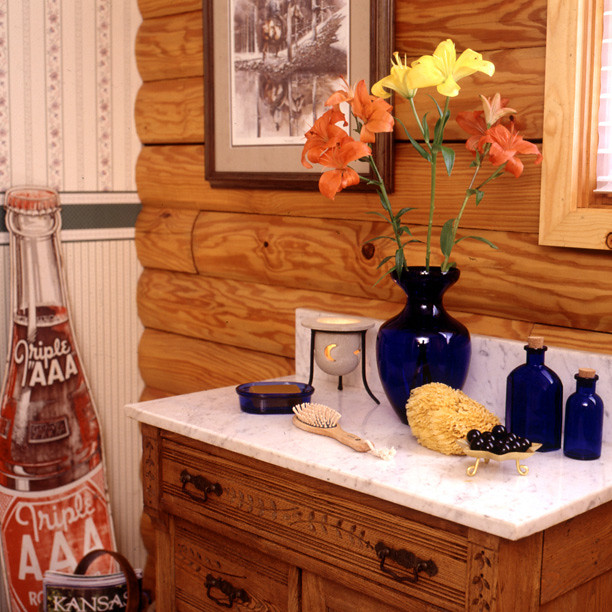In this image of a bathroom countertop, the setting exudes a rustic log cabin aesthetic. The countertop itself is not a sink but an accent surface adorned with several decorative items. The log cabin's signature wooden logs serve as a charming backdrop, enhancing the rustic ambiance of the room.

The countertop features two eye-catching cobalt blue bowls, positioned to draw attention with their vibrant color. A candle and a brush are also arranged on the surface, contributing to the countertop's cozy and functional decor. A tray holds spherical scent beads, adding a touch of fragrant elegance to the scene. 

Centrally placed on the countertop is a vase containing three artificial flowers: two bright orange blooms flanking a sunny yellow flower in the middle. To the left of the countertop, a picture frame showcases a winter scene, complementing the rustic theme with its seasonal imagery.

A striking element in the room is the large advertising sign for "Ripple Triple Triple A Cola," situated in the corner to the left of the countertop. This vintage sign adds a nostalgic touch to the log cabin bathroom. The walls are adorned with wallpaper that has both vertical and horizontal stripes, adding a layer of intricate design to the overall rustic decor.